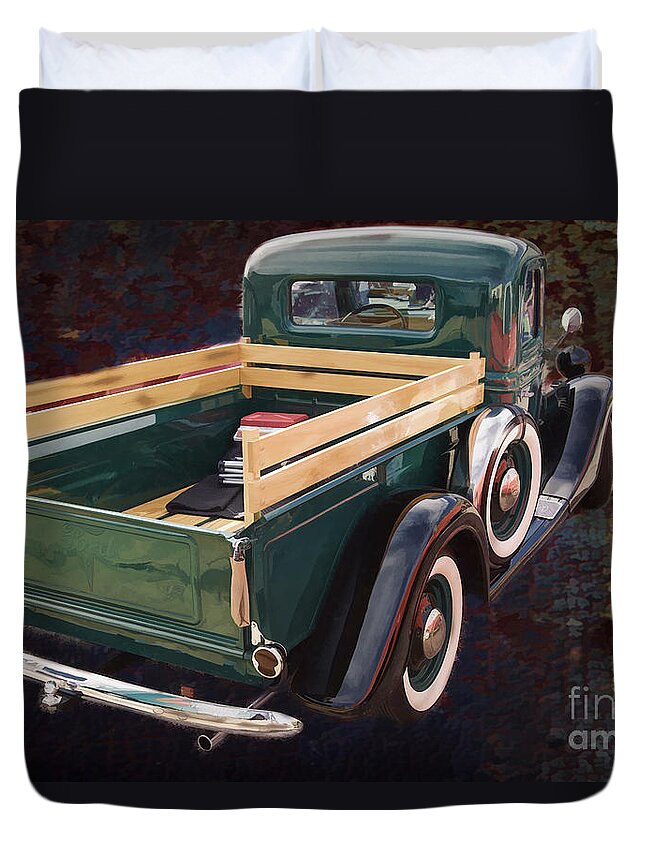This detailed painting, which appears printed on a bedspread, depicts a classic American pickup truck from the late 1940s to early 1950s. The truck, a striking dark emerald green to forest green color with varying shades, features polished chrome accents and a navy blue trim. The rear perspective of the truck showcases whitewalled tires and a shiny, highly polished chrome bumper. Inside the exposed bed of the pickup, the wooden slats create a rustic frame, holding various items like a cooler, a camp chair, a blanket, and potentially a tool kit or lunchbox. The bed itself has a wooden plank floor, enhancing the vintage aesthetic. The backdrop of the image is predominantly black, suggesting a nighttime or dimly lit setting, with hints that the painting spans a bedspread, complete with protruding pillows. The luminous quality of the truck's paint reflects a degree of outdoor light, contrasting with the otherwise dark background.